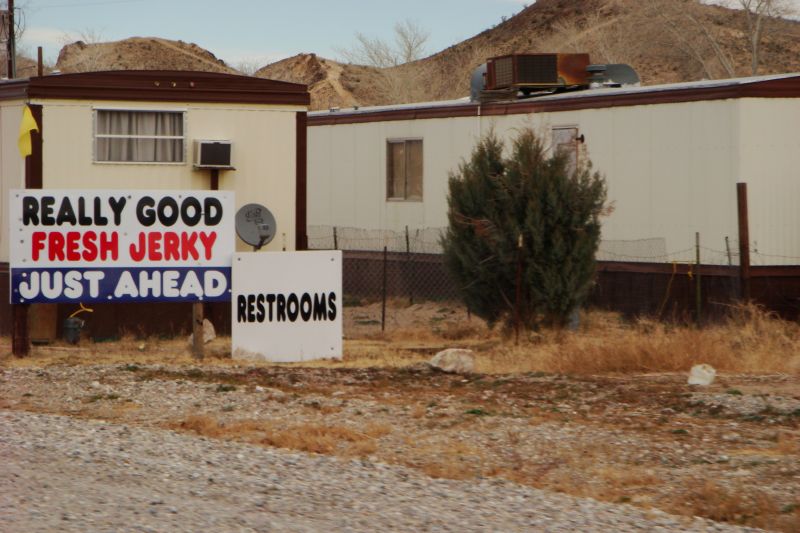The image shows a barren, outdoor setting featuring a couple of mobile homes or trailers. The primary trailer is white with a brown roof and an external air conditioning unit mounted beside its single window. Positioned in front of the trailer is a small, green, bushy tree. A prominent brown icon or possibly a speaker system sits atop this trailer. Nearby stands a series of signs: a white one with "restrooms" written in black ink, another sign which has "really good" in black, "fresh jerky" in red, and "just ahead" in white on a blue-painted bottom. A small satellite dish, possibly for TV, is attached next to the signs. There is also a yellow flag placed next to the trailer. The surroundings are characterized by dead grass and weeds, indicating a lack of irrigation. In the background, barren hills under a clear blue sky are visible, suggesting it is daytime. The entire scene gives off a sense of an arid, possibly remote area.